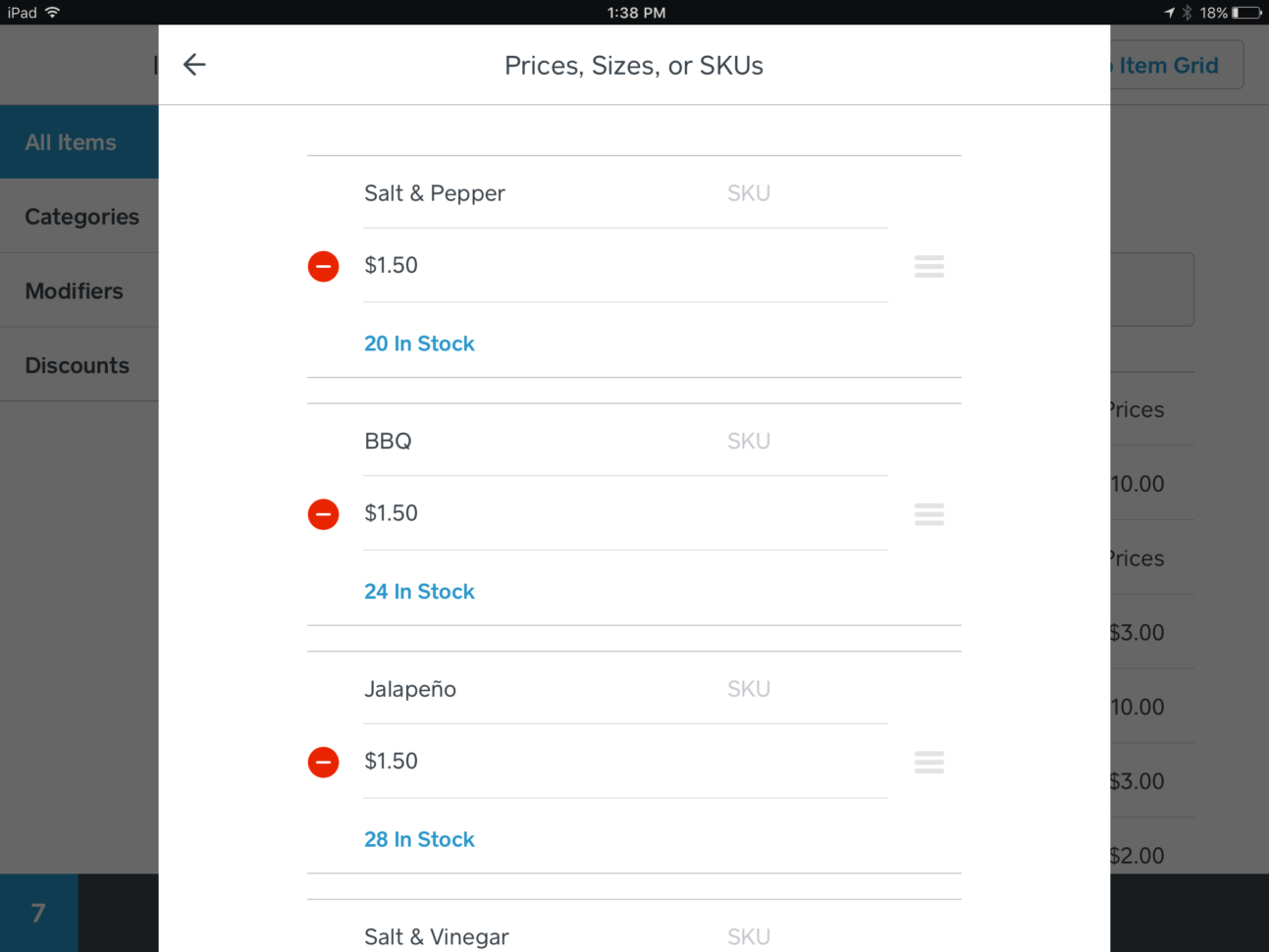The image depicts the screen of an iPad with various elements. At the top, there's a black status bar displaying the "iPad" label, a Wi-Fi symbol, the time (which is too small to be read), an unclear icon, a faint icon, and a battery indicator showing 18% charge.

Below the status bar, a grey box mainly obscured by a large white rectangle is visible. On the left side of the grey box, a blue rectangle labeled "All Items" appears. Beneath it, the term "Categories" is listed, followed by lines labeled "Modifiers," "Discounts," and others. 

On the white rectangle, there is a left-pointing arrow beside the text "Prices, Sizes, or SKUs." Under this sentence, there are several grey lines with item details:
- "Salt and Pepper, SKU" next to a circled dash, displaying a price of "$1.50," along with a blue label stating "20 in stock."
- The next section describes "BBQ, SKU" beside another red circled dash, priced at "$1.50," with a stock indication of "24 in stock."
- Finally, "Jalapeno, SKU" is itemized, accompanied by a red circled minus, priced at "$1.50," also noting it has "28 in stock."

Each item section also includes multiple grey lines, possibly indicating additional details or separations between sections.

The entire layout is a detailed snapshot of what seems to be an inventory or sales management interface on an iPad.